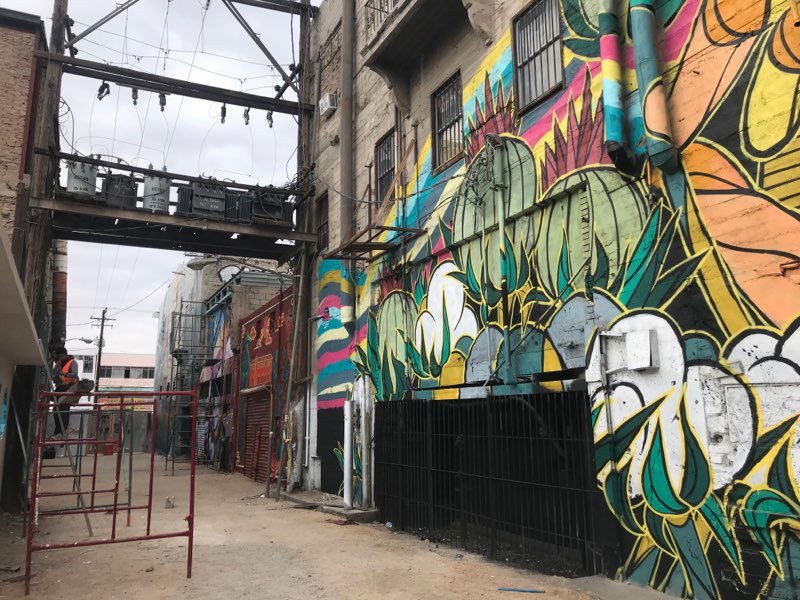The image portrays an intriguing urban alleyway, rich with cultural vibrancy and architectural diversity. To the left, an old brick building with rusty scaffolding and an orange-vested worker stands out. Between this building and another edifice, there is an alley that features a variety of graffiti art, prominently displayed on the right side. The graffiti is vividly colorful, with ornate depictions of fruits, vegetables, green cactus bulbs, and orange petals, creating a striking contrast to the gray stone facades. Below the colorful murals, black-barred windows and a black fence frame the scene. Further into the background, the buildings are less decorated, featuring muted tones of orange, blue, and tan, and topped with square roofs. Overhead, a web of wiring and some light units adorn the scaffolding. The sky above has a mix of blue and muddy grayish patches, and utility poles with visible power lines stretch into the distance. Subtle details like the red fence barriers and the tan-colored ground add to the captivating urban tapestry of this scene.